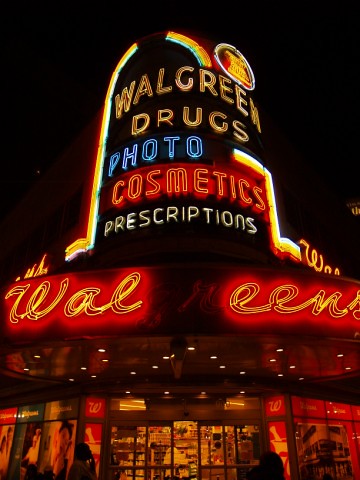This is a nighttime color photograph capturing an old-fashioned Walgreens neon sign. The sign prominently displays "Walgreen Drugs" in yellow neon, "Photo" in blue neon, "Cosmetics" in red neon, and "Prescriptions" in white neon. Below these, the name "Walgreens" is illuminated in red neon, with the 'G' and 'R' noticeably burned out. Beneath the glowing signage, the store’s storefront is visible. The automatic glass doors are positioned at the front, offering a glimpse inside where various items are displayed, though none are distinguishable due to the distance. Flanking the store’s entrance are numerous advertisements on both sides. The scene is devoid of any visible people, and the sky remains a deep, uninterrupted black, emphasizing the vibrant neon lights.